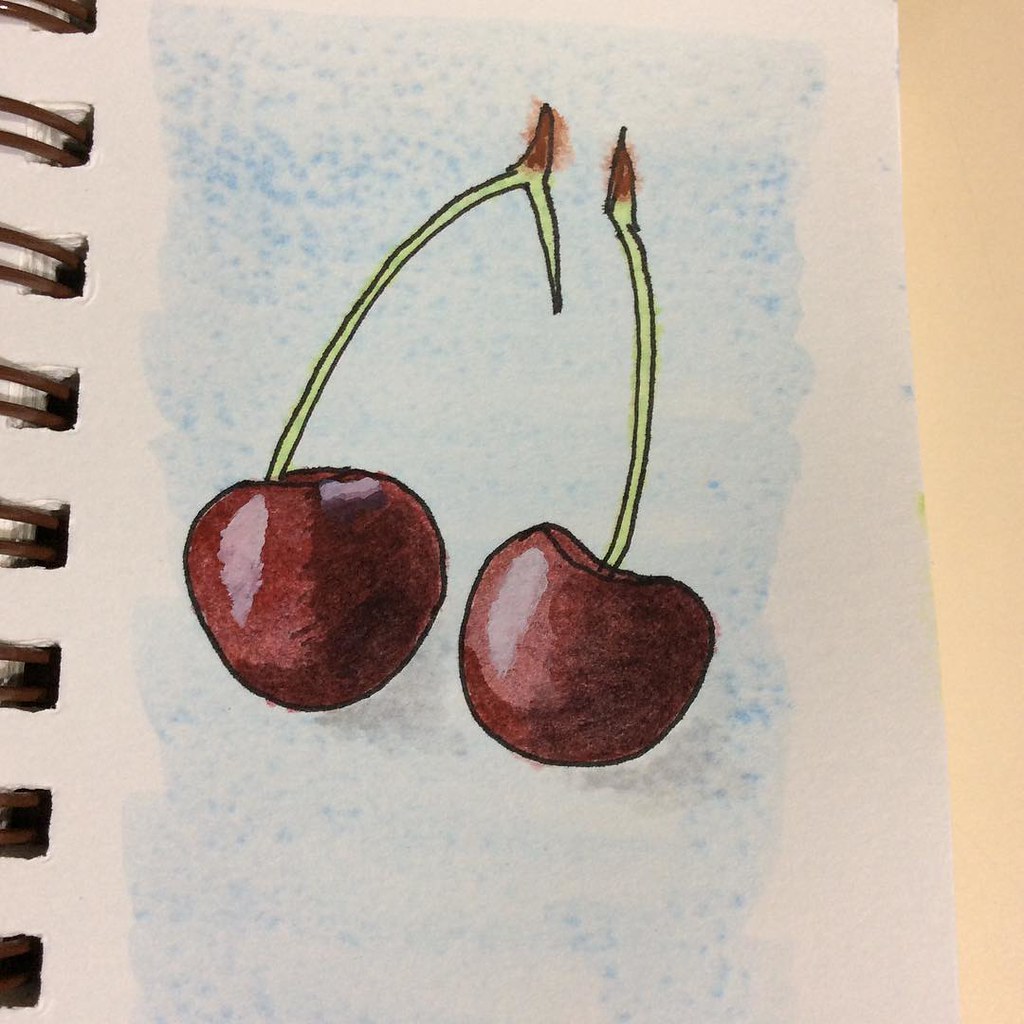In this detailed drawing from a sketchbook, identified by the black spiral rings on the left-hand side, the white paper contrasts against a peachy-colored background. The medium used appears to be watercolor, creating a blotchy blue backdrop. Centered on the page are two cherry stems, meticulously illustrated, likely with a fine-point black marker. The stem on the left is longer and light green, with a small offshoot at the top, while the right stem is singular and simpler. The cherries, almost perfectly circular except for a slightly flat top, showcase a rich, dark red hue on their shadowed right sides, transitioning to a lighter pink where the light hits, with delicate whitish-pink highlights capturing the luminosity.